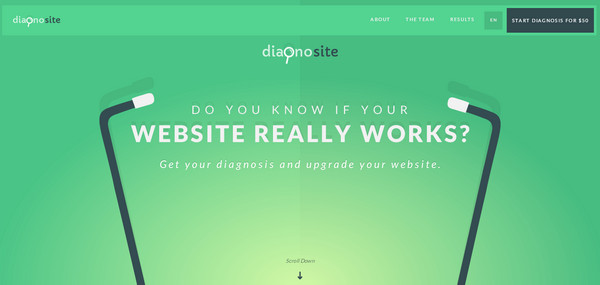**Caption:**

A mock-up of a website template for "Daya Daya Ohno". The logo, featuring a magnifying glass incorporated into the first "O" of "Ohno", is prominently displayed in the upper left corner and again in the center below the header. The menu header on the right includes navigation options: "About", "The Team", "Results", "Start Diagnostics for $10", and an additional button that's difficult to discern. Central to the design is a simplistic graphic resembling a stethoscope made from two angled gray bars with white tips. The main promotional text, "DO YOU KNOW IF YOUR WEBSITE REALLY WORKS?", is displayed in large capital letters with an upward shadow effect. Below this, the text encourages users to "Get your diagnosis and upgrade your website", with an option to scroll down. The overall color scheme of the website is seafoam green, complemented by a graded yellowish glow in the center area beneath the main text. This basic design serves as a starting point for conceptualizing a potential real website, though it remains incomplete with no visible URL.